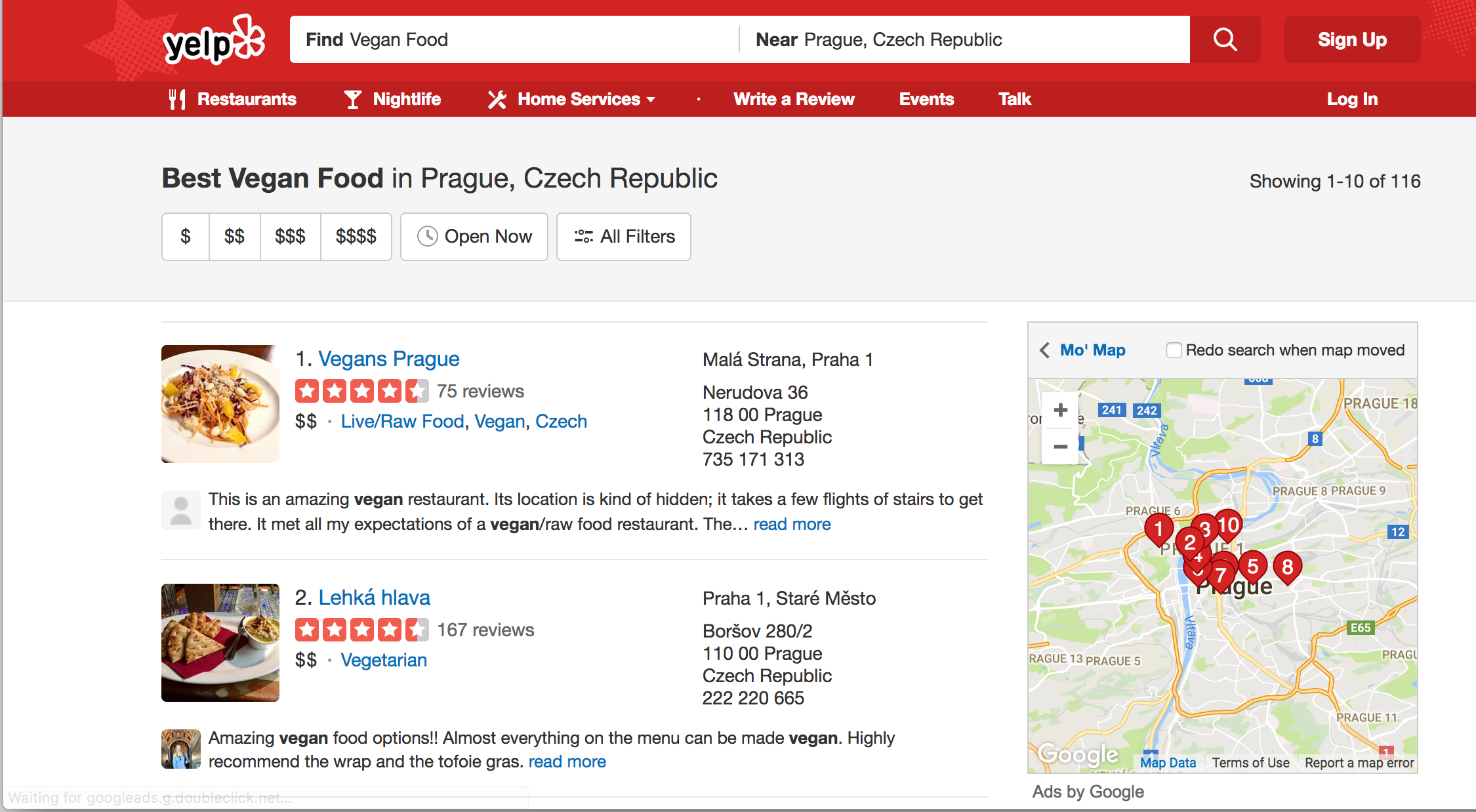**Detailed Caption: Desktop Screenshot of Yelp Page Showing Vegan Food Options in Prague, Czech Republic**

This desktop screenshot captures a user navigating Yelp's website, specifically searching for vegan food in Prague, Czech Republic. The interface displays the iconic Yelp name and logo at the top left, alongside a search bar populated with "find vegan food near Prague, Czech Republic." Adjacent to the search bar, options to “Sign Up” and “Log In” are visible.

Below these options, a horizontal menu showcases Yelp’s main categories: Restaurants (symbolized by fork and knife), Nightlife (indicated by a martini glass), Home Services (illustrated with a wrench and another tool), as well as links for Writing a Review, Events, and Talk, alongside another “Log In” link.

The page prominently reads “Best Vegan Food in Prague, Czech Republic.” Users can refine their search using filters for price ranges (from $ to $$$$), open hours (Open Now), and more (All Filters). A summary indicates that the current view is displaying results 1 to 10 out of 116.

At the bottom right, there is a clustered map displaying 10 pinned locations, though only two specific results are visible on the screen.

1. **Vegan's Prague**
   - **Rating**: 4.5 stars out of 5
   - **Reviews**: 75
   - **Price Scale**: $$ (2 out of 4)
   - **Cuisine**: Live/Raw Food, Vegan Czech
   - **Address**: Mala Strana, Praha 1, Nerudova 36, 11800 Prague, Czech Republic
   - **Phone**: +420 735 171 313
   - **Description**: A hidden gem requiring a few flights of stairs to access, Vegan's Prague meets all expectations for a vegan/raw food restaurant. The description invites users to "read more" for additional details.

2. **Lehká Hlava**
   - **Rating**: 4.5 stars out of 5
   - **Reviews**: 167
   - **Price Scale**: $$ (2 out of 4)
   - **Cuisine**: Vegetarian
   - **Address**: Praha 1, Staré Město, Borsov 280/2, 11000 Prague, Czech Republic
   - **Phone**: +420 222 220 665
   - **Description**: Offering a multitude of vegan options, almost everything on the menu can be made vegan. Notable recommendations include the wrap and the Tofoigras. Further details are available to "read more."

This detailed breakdown reflects a user’s quest for vegan dining options in Prague, highlighting specific establishments and their key information on Yelp’s platform.